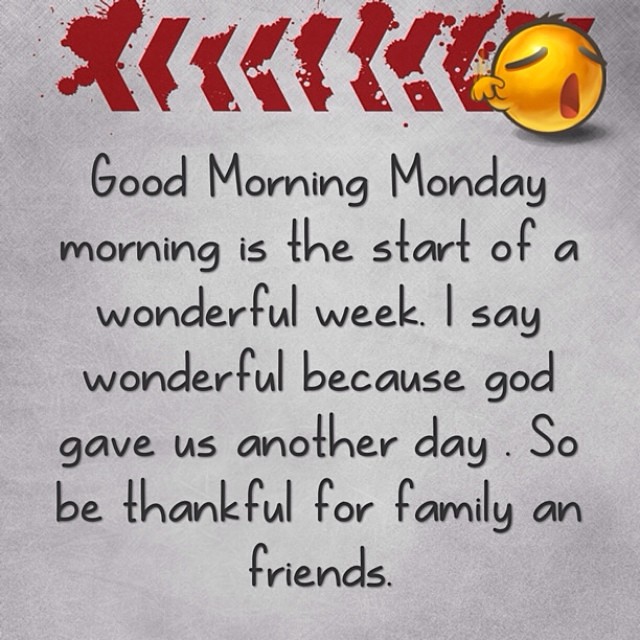The image features a light gray background with a prominent motivational message designed for social media or a card. Centered in black text, the message reads, "Good morning Monday. Morning is the start of a wonderful week. I say wonderful because God gave us another day. So be thankful for family and friends." Above this text, towards the top, is a red logo or design consisting of small, wide arrows pointing to the left. Some arrows show smudges or pieces missing, and they are accented with splotches of red and gray, almost giving a distressed effect. In the top right corner, there's a yellow emoji with eyes closed and mouth wide open, suggesting a yawn, with a small hand to the left of the face. The colors in the image include gray, red, yellow, pink, and tan. The overall style is motivational and positive, likely intended to encourage viewers to start their week with gratitude.